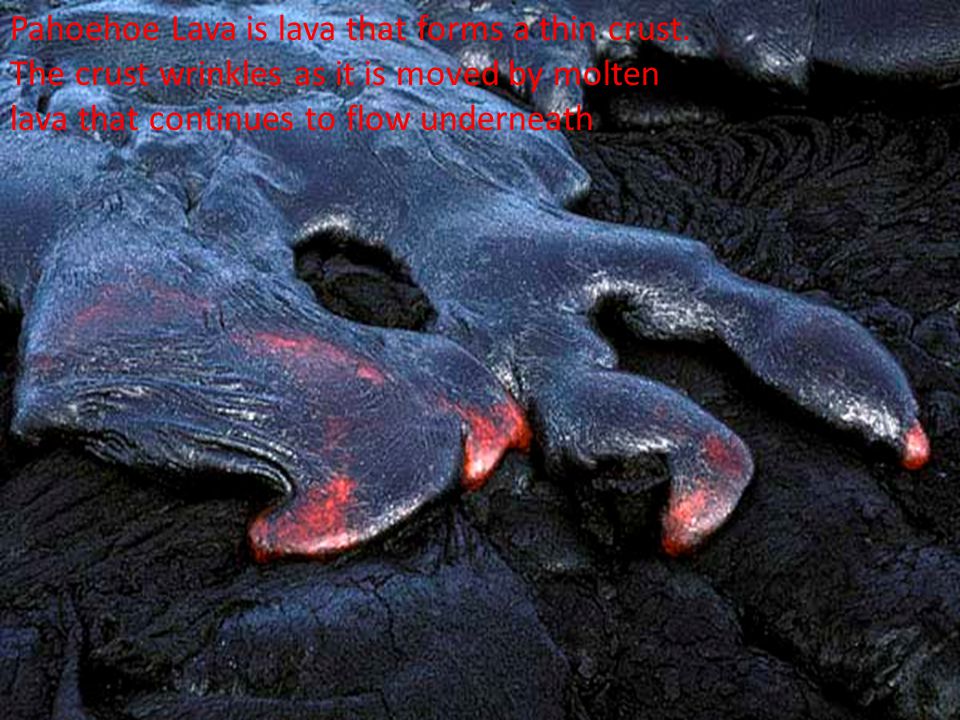The image depicts Pāhoehoe lava, characterized by its thin, glossy crust that forms as the molten lava cools and hardens. The crust shows intricate wrinkles and folds as it is continually pushed by the flowing molten lava beneath. The outer surface of the lava is black, but fissures and fresh lava veins reveal glowing, ember-like red sections within. These visible rifts, including a central crack that splits into a V formation with vivid red tips, highlight the active nature of the underlying molten lava. The overall scene captures the dynamic contrast between the dull, cracked crust and the radiant, liquid lava, with the shinier molten areas reflecting light and appearing wet compared to the dark, solidified regions. White specks glinting in the molten sections add to this visual distinction, emphasizing the flow and movement of the lava.